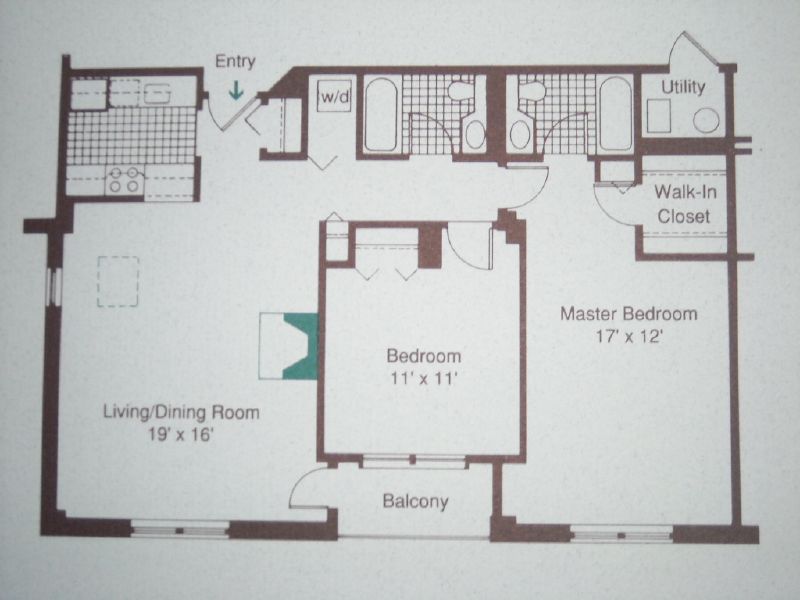The floor plan features an entryway located in the top left corner. Upon entering, you proceed directly ahead to a spacious combined living and dining area measuring 19 by 16 feet. Immediately to the left of the entry, you'll find a washer and dryer, and on the right, there is a bedroom measuring 11 by 11 feet. Continuing straight down the hallway, you'll reach a door that leads to the master bedroom on the right, which spans 17 by 12 feet and includes a walk-in closet. Additionally, there is a separate utility room accessible from outside, ideal for storage. The bottom of the floor plan showcases a balcony attached to a middle bedroom. The layout also includes several windows, although their specific type—whether sliding doors or standard windows—remains unclear. Overall, the design offers a spacious and functional living environment, with well-thought-out rooms and utility spaces.